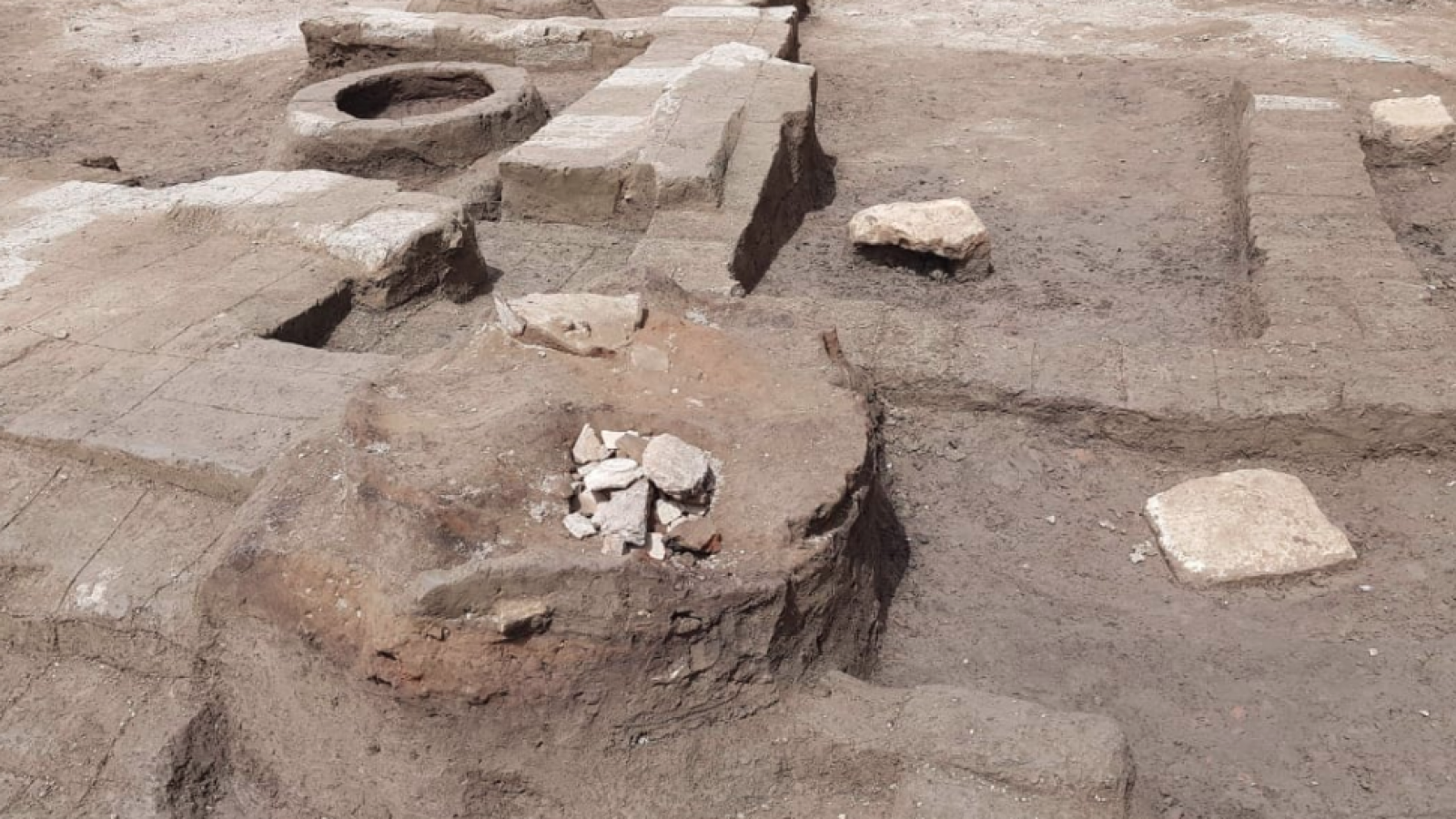This digital photograph captures a meticulously excavated archaeological site, likely an ancient city. The scene, viewed from a slightly elevated position, reveals the weathered remnants of large stone structures and foundations. The dominant hues are earthy browns and grays, indicating dried ground and possibly the presence of clay or chalk. In the upper left, a series of stone steps ascend toward a prominent circular pit, possibly an ancient kitchen or kiln. Scattered bricks and pieces of rock frame the partially uncovered site, which is largely free of rubble. In the center, near the bottom of the frame, stand broken bits of what might have once been a pillar or a storage structure, hinting at the site's storied past.